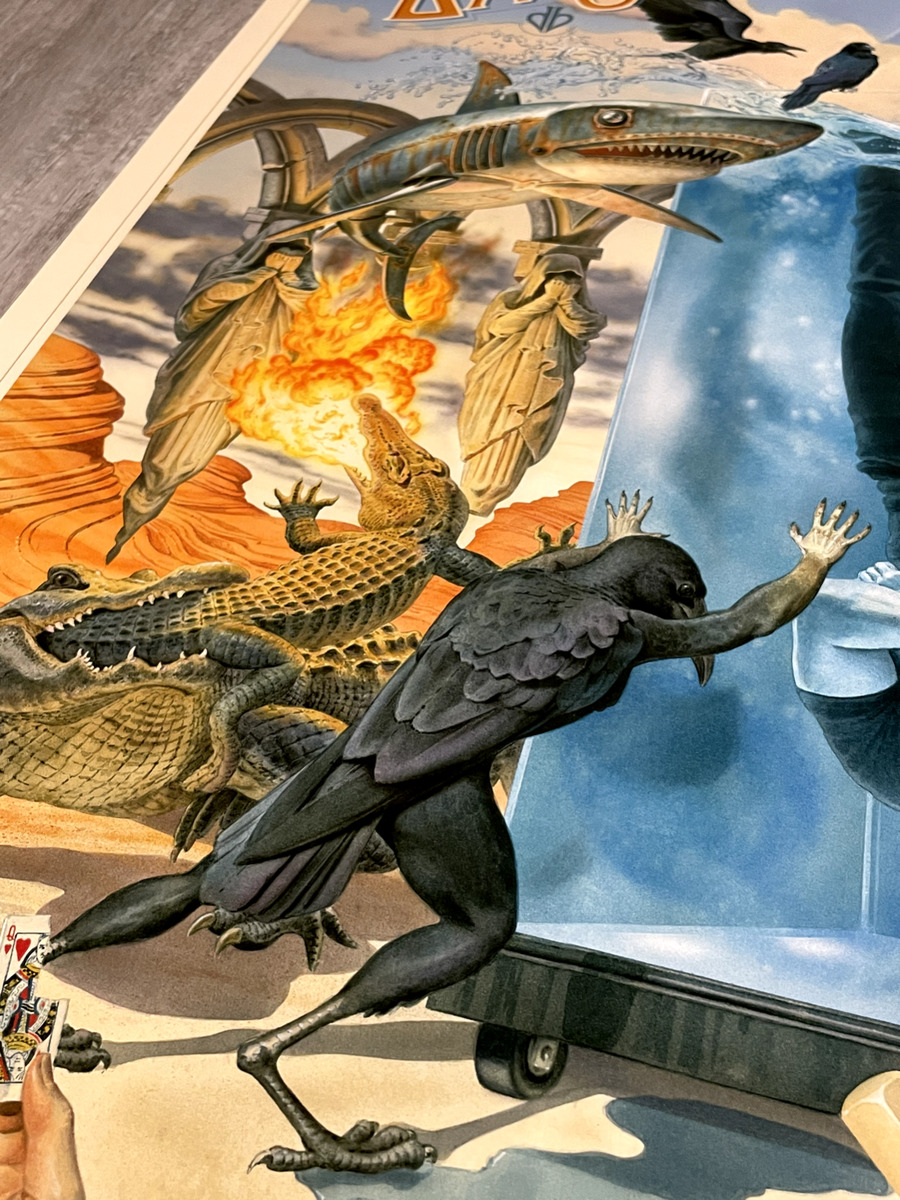This is an image of a detailed illustration resting on a gray tabletop. The illustration features a surreal and futuristic scene. Dominating the scene, a large bird resembling a raven or crow, but with human-like arms and hands, is pushing a glass cart with small wheels. The cart, seemingly filled with water, contains an upside-down man. To the left, an alligator is seen devouring another alligator that is breathing fire into a landscape reminiscent of the red rocks of Utah or Arizona. Above, a shark flies through the sky adding to the peculiar nature of the scene. In the foreground on the bottom left, a person's hand is holding a Queen of Hearts playing card with the top right corner torn off. The overall composition includes various images and elements, creating a fantastical and bizarre tableau.